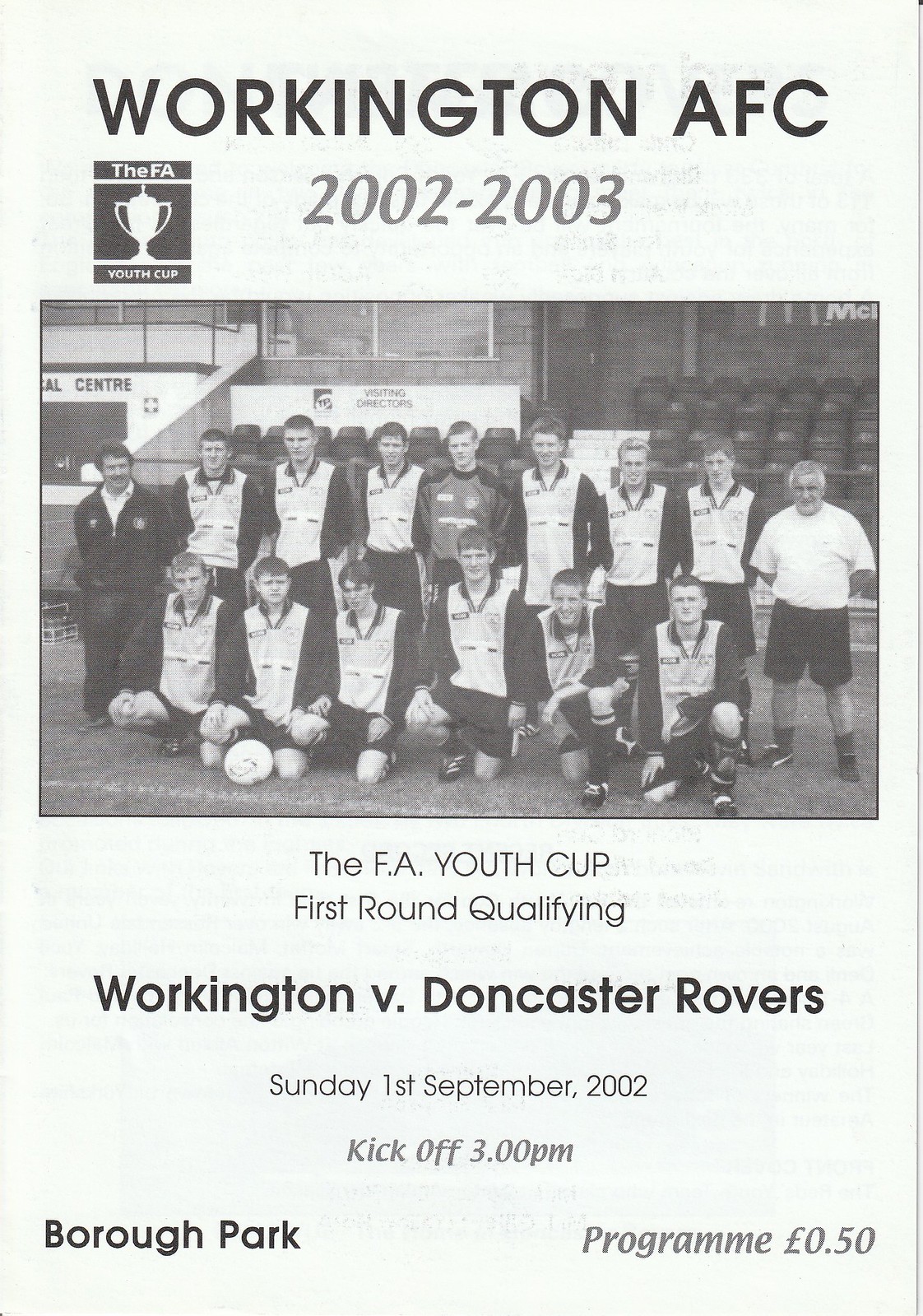This is the cover of a black and white program for the Workington AFC soccer team from the 2002-2003 season. At the top, it boldly states "Workington AFC 2002-2003." In the upper left corner, there's a logo depicting a cup with the words "FA Youth Cup" above and below it. Dominating the center of the program is a group photo of the team in their soccer uniforms, arranged in two rows: those in the back row are standing, while those in the front row are kneeling with a ball placed in front of them. Flanking the team are two men, possibly the coach and an assistant; one is wearing a white shirt and shorts, the other a zipped-up jacket. Below the team photo, the program details the event: "FA Youth Cup First Round Qualifying," followed by "Workington vs. Doncaster Rovers," the date "Sunday, 1st September 2002," and the kickoff time "3pm." At the bottom, the location is noted as "Borough Park" on the left, and the price, "50 cents," is printed on the right-hand side.